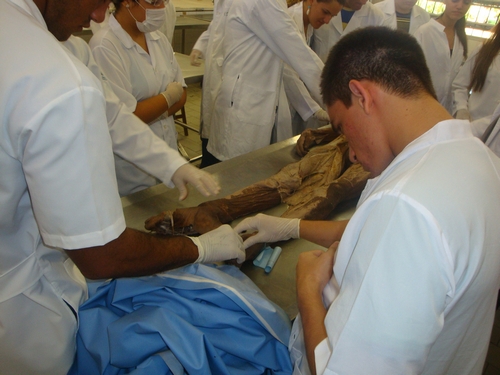In this detailed image, a group of eight to nine individuals, a mix of men and women, are gathered around a steel table or slab wearing lab coats, white outfits, and surgical gloves, intently analyzing a motionless and very dry, brown corpse. Two men, one on the left and one closer to the bottom of the photo, are shown touching the foot of the deceased, with their gloved hands, while several other individuals in the background are examining the upper part of the body. The corpse's appearance suggests it might have been burned, as indicated by its charred and untattered state. A blue smock or cover is crumpled at the bottom of the image, hinting that it has recently been removed to unveil the remains. On the left side, one person is notably wearing a surgical mask, and there is a general atmosphere of focused yet somber examination among the group, akin to a medical study or forensic investigation.